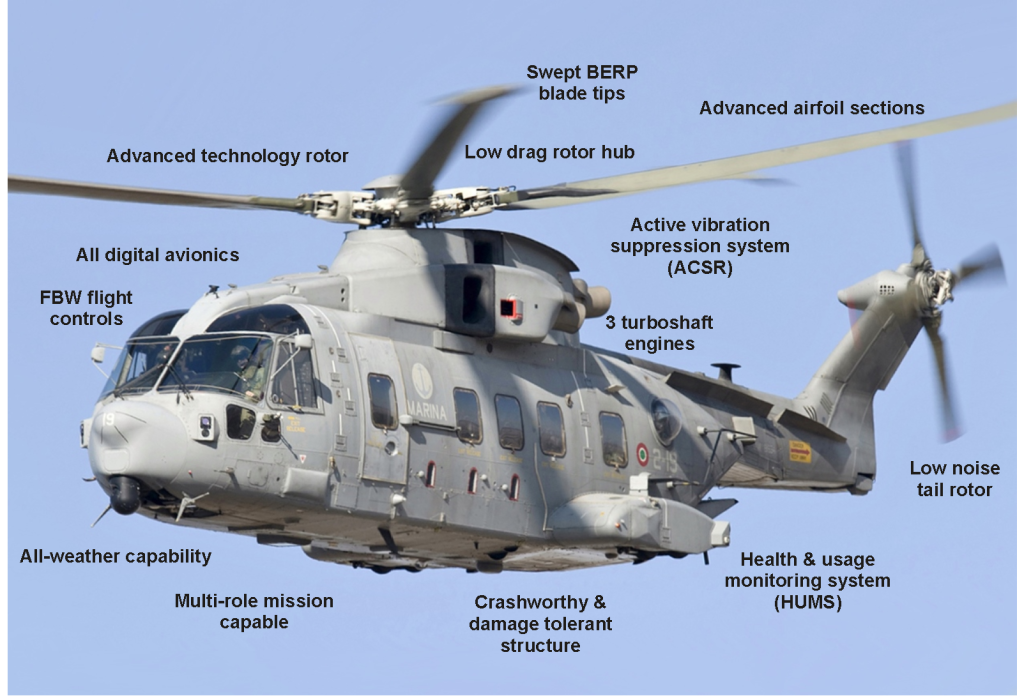This detailed photorealistic image portrays a gray military helicopter, resembling the length of a small bus, and is displayed against a uniform light blue background. The helicopter, which might be identified as a Chinook, features both a top and rear rotor, with the top rotor appearing blurred as if caught in motion. The aircraft displays the word "Marina" near the front, accompanied by a picture of an anchor, suggesting naval use, and bears the number 219 along with a green-centered bullseye.

The helicopter's pilot, wearing military camouflage and a helmet, is visible through one of the six windows (including the cockpit). The illustration labels various advanced technologies in black text around different parts of the helicopter, boasting features like "Advanced Airfoil Sections," "All Digital Avionics," "FBW Flight Controls," and "Crash-Worthy and Damage Tolerant Structure." Additionally, highlighted technologies include "Swept BRP Blade Tips," "Advanced Technology Rotor," "Low Drag Rotor Hub," "Active Vibration Suspension System," "Three Turboshaft Engines," "Health and Usage Monitoring Systems (HUMS)," "Low Noise Tail Rotor," and "All Weather Capability." This meticulous labeling appears to emphasize the helicopter's multi-role mission capabilities and the sophisticated technology it incorporates.